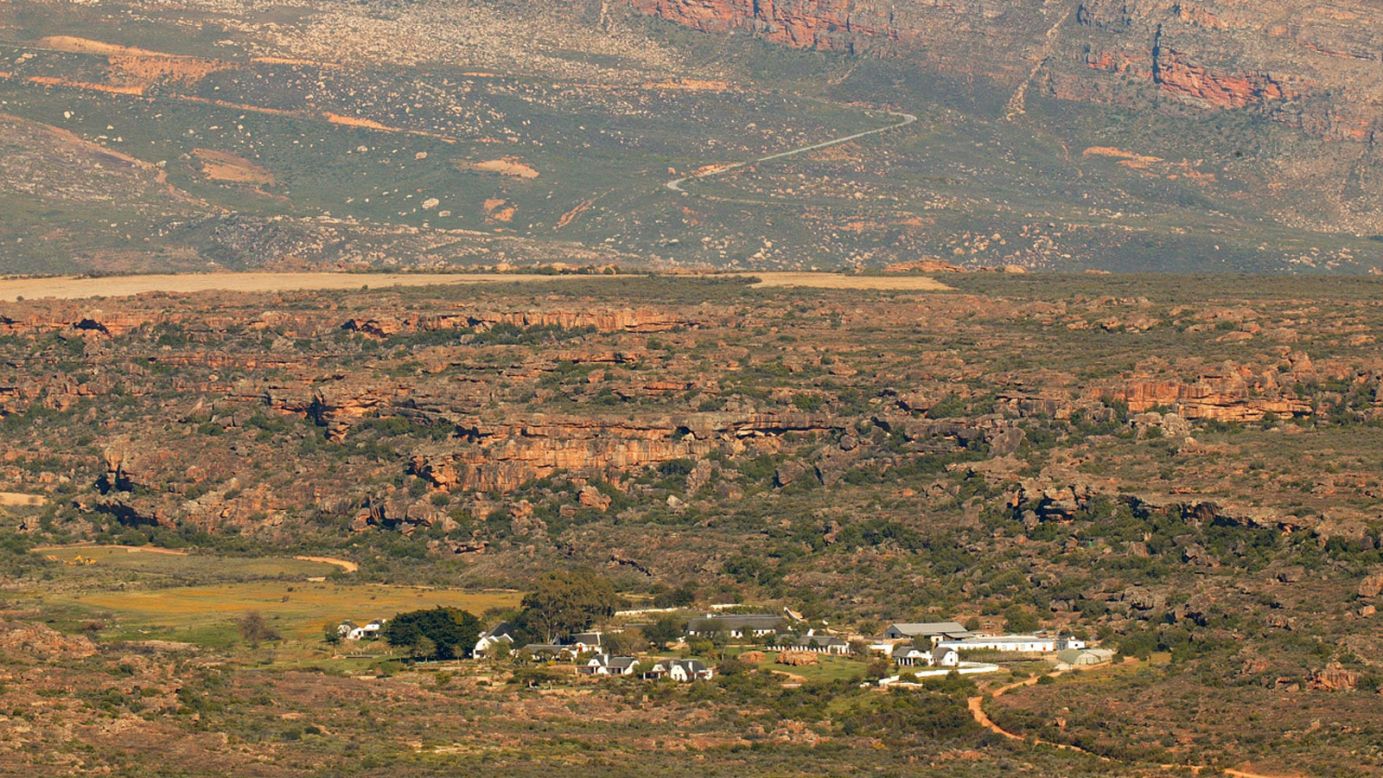The image features a stunning aerial view, likely taken from a high vantage point or drone, of a vast desert landscape in the southwestern United States. Dominating the foreground are light brown grounds intermixed with patches of green vegetation. Nestled in the lightly colored arid terrain is a small collection of white, ranch-style houses with gray roofs, forming a tiny town or settlement. The area extends horizontally, revealing more brown and green mixed terrains. On the left side, there is a noticeable patch of greener land, contrasting with the expansive dry surroundings. To the top right, the landscape transitions into rocky, canyon-like mountainous structures. The overall scene evokes a sense of solitude and quiet beauty, capturing the essence of a place poised between desert barrenness and the occasional burst of greenery.